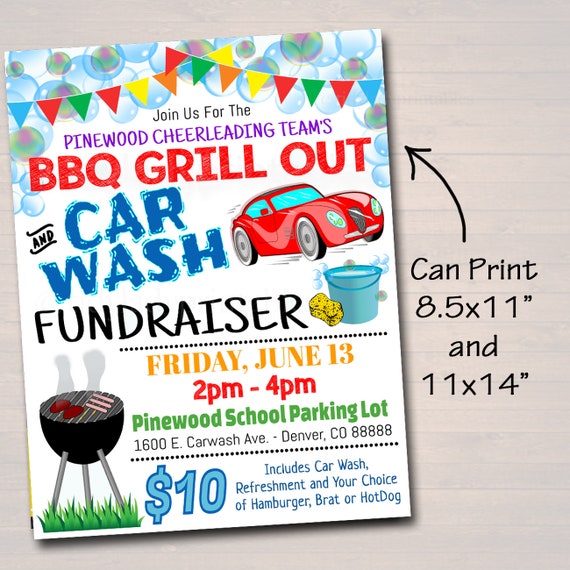A colorful and lively poster is showcased against a plain beige background. The poster is adorned with festive balloons and party flags at the top, inviting viewers to "Join us for the Pinewood Cheerleading Team's Barbecue Grillout and Car Wash Fundraiser." The event is scheduled for Friday, June 13th, from 2 to 4 p.m. at the Pinewood School parking lot in Denver, Colorado. For $10, attendees can enjoy a car wash, refreshments, and their choice of a hamburger, brat, or hot dog. The bottom of the poster includes additional details in black lettering, noting that the poster is available for printing in sizes 8.5 by 11 inches and 11 by 14 inches.